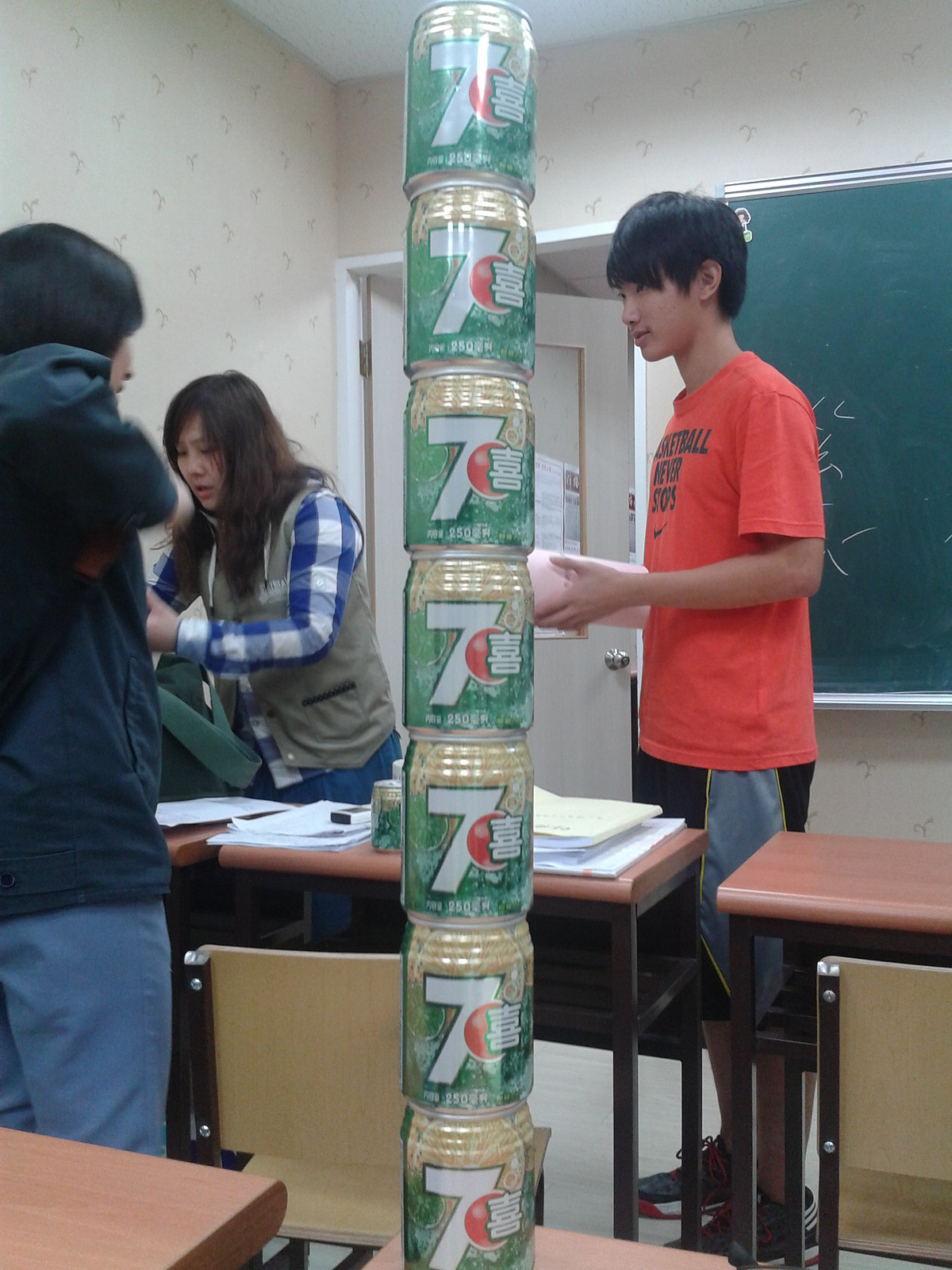A vibrant photograph, capturing a moment in a Japanese classroom, takes center stage with a stack of seven uniquely designed 7-Up cans prominently positioned on one of the desks. These cans feature a modern design with a red ball in front of a white '7' and Japanese characters, set against a silver background. In the background, the classroom’s rows of desks and chairs are visible, along with a green chalkboard on the upper right. The classroom door, white with a glass panel, is ajar, swinging outward into the hallway.

Three figures populate the scene: On the left, a girl with straight black hair, dressed in blue pants and a dark blue top, is partially visible in profile as she converses with a boy. The boy, standing towards the right, sports an orange t-shirt with some writing and holds a rolled-up piece of paper. His attire includes basketball-style shorts, blue with a light blue panel on the side. Meanwhile, a girl with a white and blue plaid long-sleeved shirt and an olive green vest sits opposite the first girl, seemingly engaged in placing something into her backpack. Their casual interactions add a dynamic, everyday feel to the academic setting.